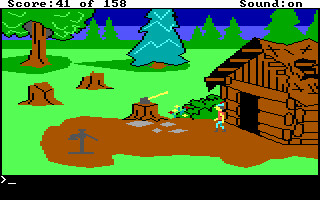This detailed depiction offers a glimpse into a vintage, pixelated video game screenshot. A purple-hued sky serves as the backdrop, alternating between light and dark purple tones. Along the horizon, several green trees stretch across, creating a stark contrast against the sky. The landscape features a lush green field interspersed with three cut tree stumps. One of these stumps, placed centrally, holds an ax embedded in its top.

To the scene’s lower right, a log cabin stands, constructed from brown logs. The cabin, shadowed beneath its left roofline, displays an open black door from which a cartoon character, depicted in a blue shirt and blue jeans, steps out onto a dirt walkway. This figure, moving leftward, encounters a bush positioned directly in front of the cabin.

In the middle ground, another distinctive feature is a blue pine tree adorned with zigzag lines, potentially mimicking Christmas lights. A traditional water pump is stationed at the end of the visible dirt path leading from the cabin. Along the bottom of the image, a black strip spans, with an arrow symbol and an underscore located at the lower left corner, emphasizing the gameplay elements present. The top of this screen reads "Score 41 of 158" on the left, and "Sound On" on the right, framing this nostalgic, interactive scene.